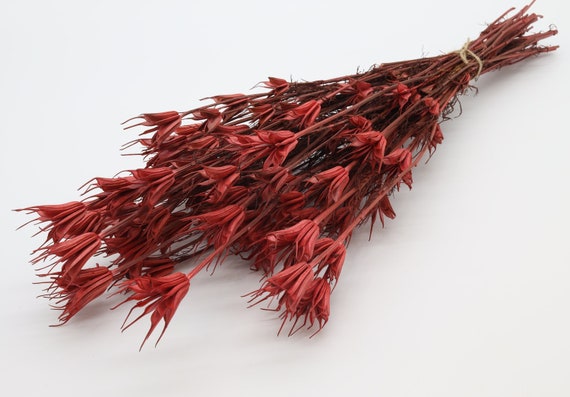This close-up, landscape-oriented color photograph vividly captures a tightly bundled bouquet of dried flowers laid diagonally against a light gray background. The bundle, comprising about 15 to 20 stems, is securely fastened near the bottom with a piece of thin, brown string. The flower heads, with their dark red, dried petals featuring multiple protruding points, are oriented towards the top left corner of the image, while the bound stems extend towards the top right. The stems exhibit a gradient coloration, transitioning from light orange at the top to a darker brown near the bottom, enhancing their desiccated appearance. The overall composition underscores the rustic beauty of the dried flowers, blending the reddish-brown hues of the blossoms with the brown of the stems in a coherent and visually pleasing manner.